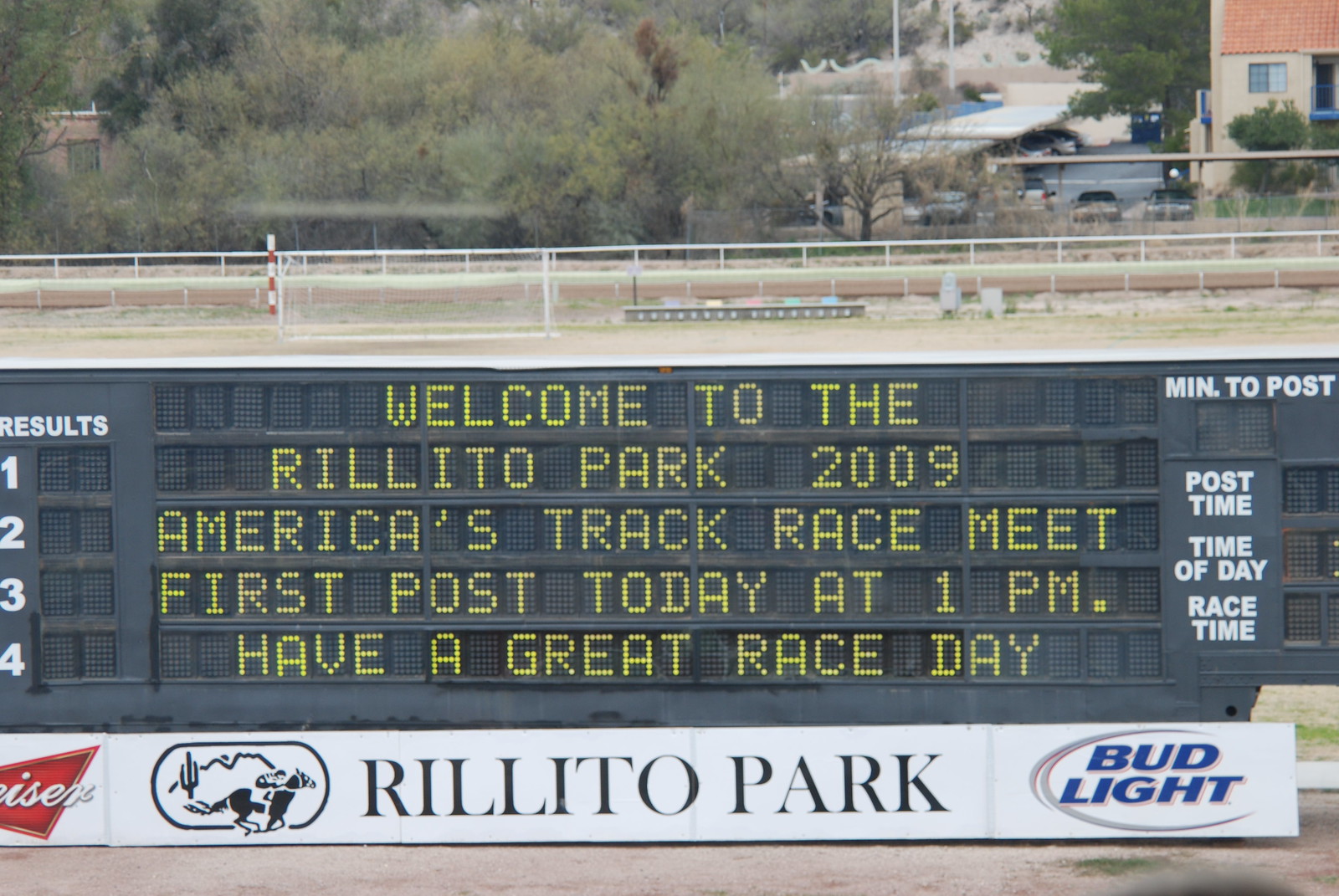This vivid color photograph captures a scene at an outdoor horse racing venue. Dominating the foreground is a large black digital scoreboard adorned with bright green lettering that reads, "Welcome to the Rillito Park 2009 America's Track Race Meet. First post today at 1pm. Have a great race day." Below this message, the scoreboard also displays "Rillito Park" and is flanked by logos for Budweiser and Bud Light, indicating sponsorship. The board further displays various racing details such as "Minutes to post," "Post time," "Time of day," "Race time," and the "Results 1, 2, 3, 4." Behind the scoreboard, a dirt horse racing track is bordered by a white fence, with lush green trees lining the background, adding a natural frame to the scene. A yellow house with a brown roof is visible in the distance, highlighting the rustic charm of the location. The overall composition emphasizes the excitement and charm of a race day at Rillito Park.